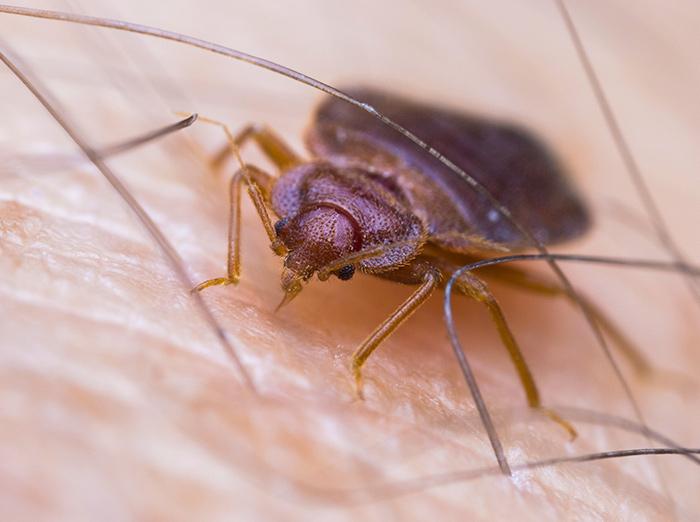This highly magnified image prominently features a bug directly in the center, located on someone's skin. The skin's intricate details are clearly visible, showing fine hairs and lines typical of human skin. The insect, which might be a cockroach, tick, or stink bug, is primarily a blend of beige, yellowish, amber, lighter brown, reddish, and black hues. The bug is positioned such that it appears to be looking towards the bottom left corner of the image. Its six legs and identifiable features make it unmissable, with the potential pointy head indicating readiness to bite. This close-up, detailed texture suggests a deliberate setting, perhaps for a documentary on insects, with the subject potentially having volunteered for this intriguing capture.